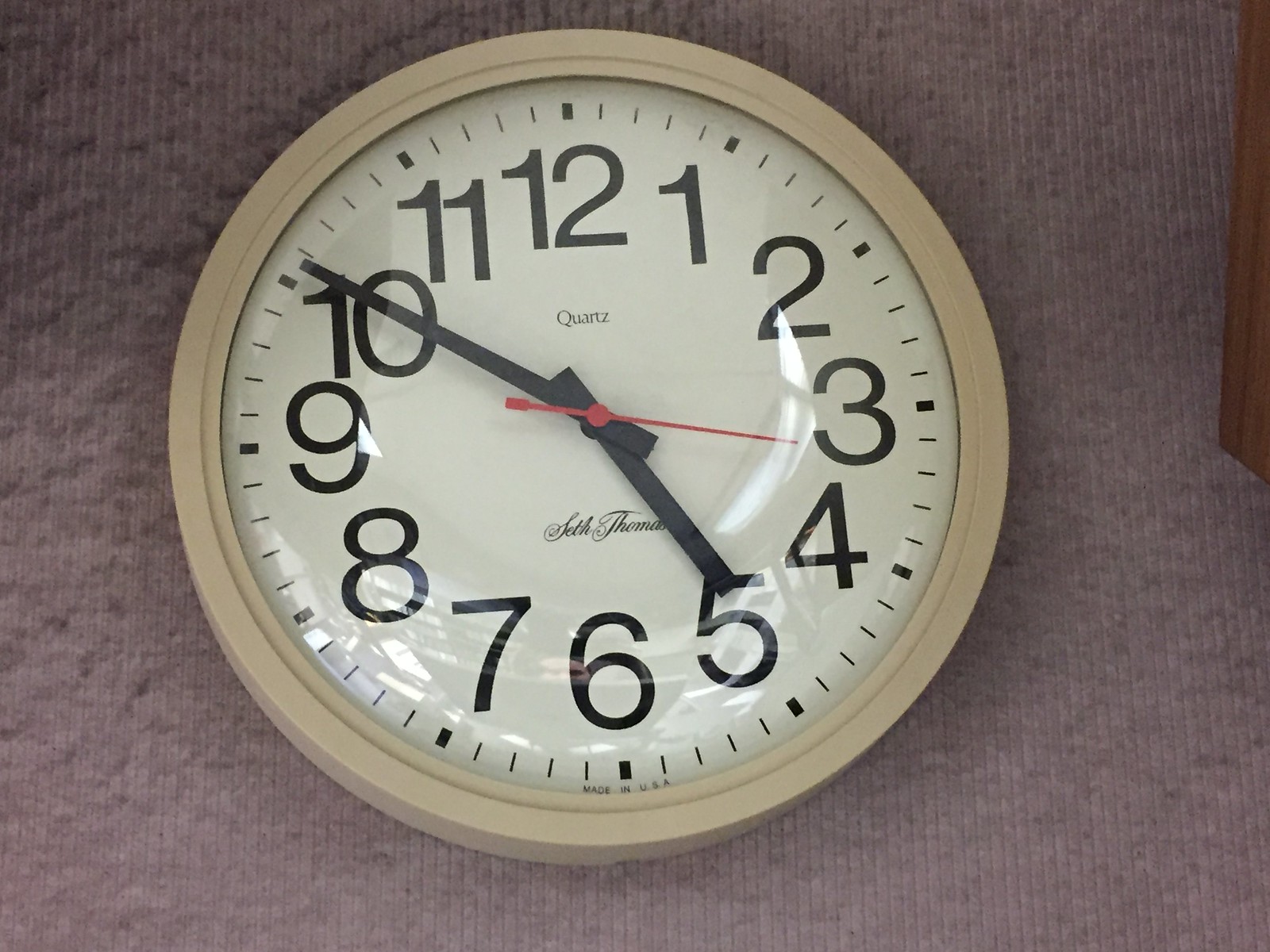This photo captures a detailed close-up of a round wall clock set against a textured background that appears to be a mauve or lavender cloth, possibly a carpet or rug. The clock features a beige circular frame with a white face. Large black numerals from 1 to 12 are clearly marked, with smaller dashes in between each number, creating a complete ring around the clock. The time displayed is approximately 4:51. The hour and minute hands are black, while the second hand stands out in red. Above the hands, the word "Quartz" is printed, and below, the brand name "Seth Thomas" is elegantly written in cursive. In the top right corner of the image, part of a wooden object, likely a piece of furniture, slightly intrudes into the frame, adding an additional element to the composition.